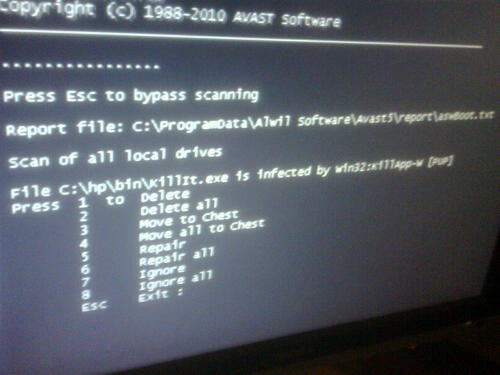This photo captures a partial view of a computer monitor displaying a screen within a DOS program. The screen is primarily a dark, washed-out black with white text. The top of the screen shows the text "Copyright (C) 1988-2010 AVAS Software." Below this, there is a line followed by several dots. A message instructs the user to "Press ESC to bypass scanning," and beneath it, there is a "Report file" path partially visible, starting with "C:\ProgramData\" and ending in ".txt." This is part of a scan report of all local drives, identifying an infected file beginning with "C:\HB\BIN." The screen provides several actions the user can take by pressing corresponding numbers: "1 to delete, 2 to delete all, 3 to move to chest, 4 to move all to chest, 5 to repair, 6 to repair all, 7 to ignore, 8 to ignore all," with "ESC to exit." The image details a scanning process of local drives to identify and manage infected files using various options.